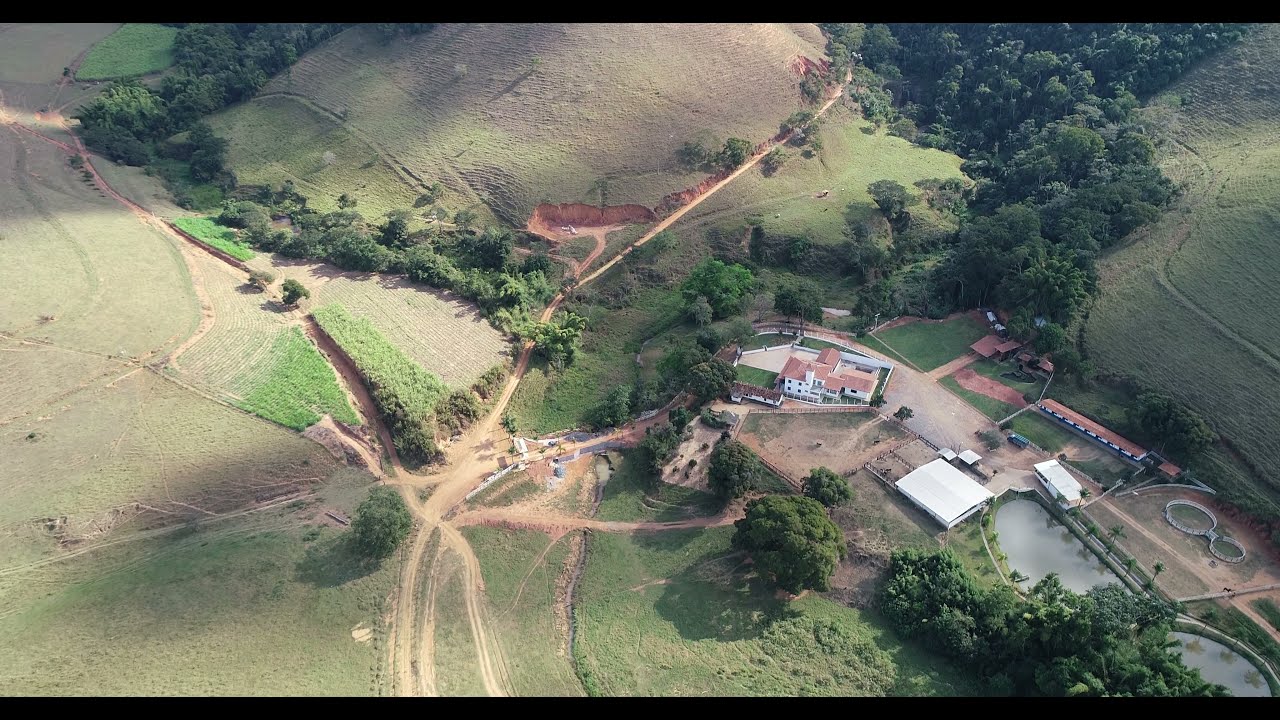The aerial image captures a sprawling estate set amidst rolling hills and a blend of grassy and wooded areas. The landscape features a network of interconnecting dirt roads radiating from a central larger patch, resembling an octopus with its tentacles stretched out. To the right of center, there is a stately white manor with a prominent red roof, flanked by several other structures. These include a long building with a red roof, possibly for stables, and a perfectly square building with a white roof. The property includes a large manmade pond surrounded by palm trees and multiple smaller buildings, some bordering the woodland edge. The right side of the image displays a balanced mix of grass and trees, while the left side is more predominantly grassy. Overall, the estate is well-integrated into the undulating topography, connected by dirt roads that extend into various parts of the property and beyond into fields and forests.